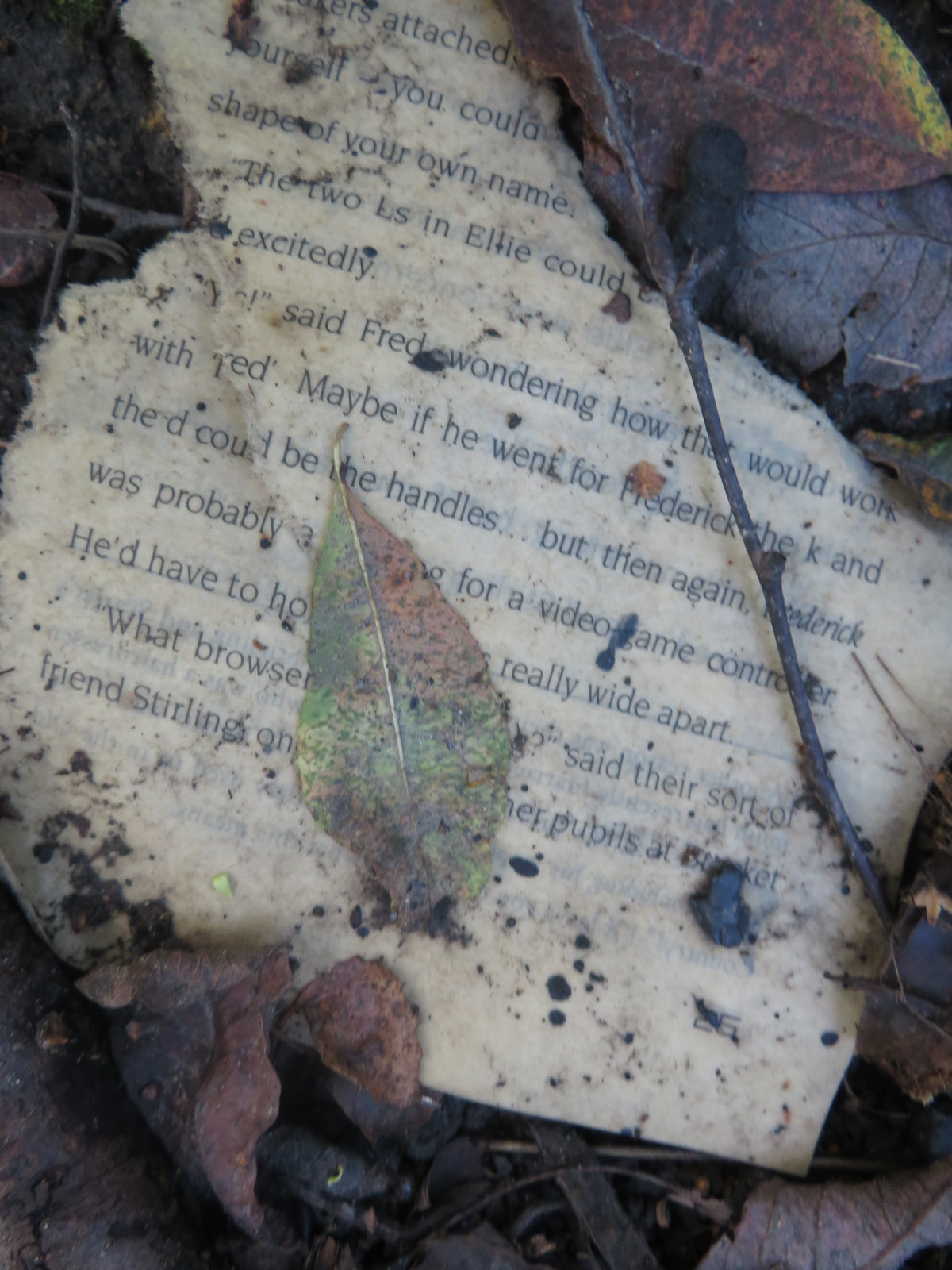In this outdoor photograph, a partially burned and torn page lies on a muddy ground, surrounded by fallen leaves, a few stones, and small twigs. The scene includes various colors, such as shades of brown, black, off-white, green, orange, and yellow, highlighting the autumnal decay. The page, which seems to have been torn out of a book or novel, is covered in ash and depicts text fragments with phrases like "Fred wondered how that would work" and "Frederick was probably." One leaf, brown and green with a hint of yellow in the upper corner, obscures part of the text, while the rest of the words are disrupted by debris and damage. The photograph captures a moment of literary destruction against a backdrop of nature's detritus, suggesting an environment that is both weathered and abandoned.